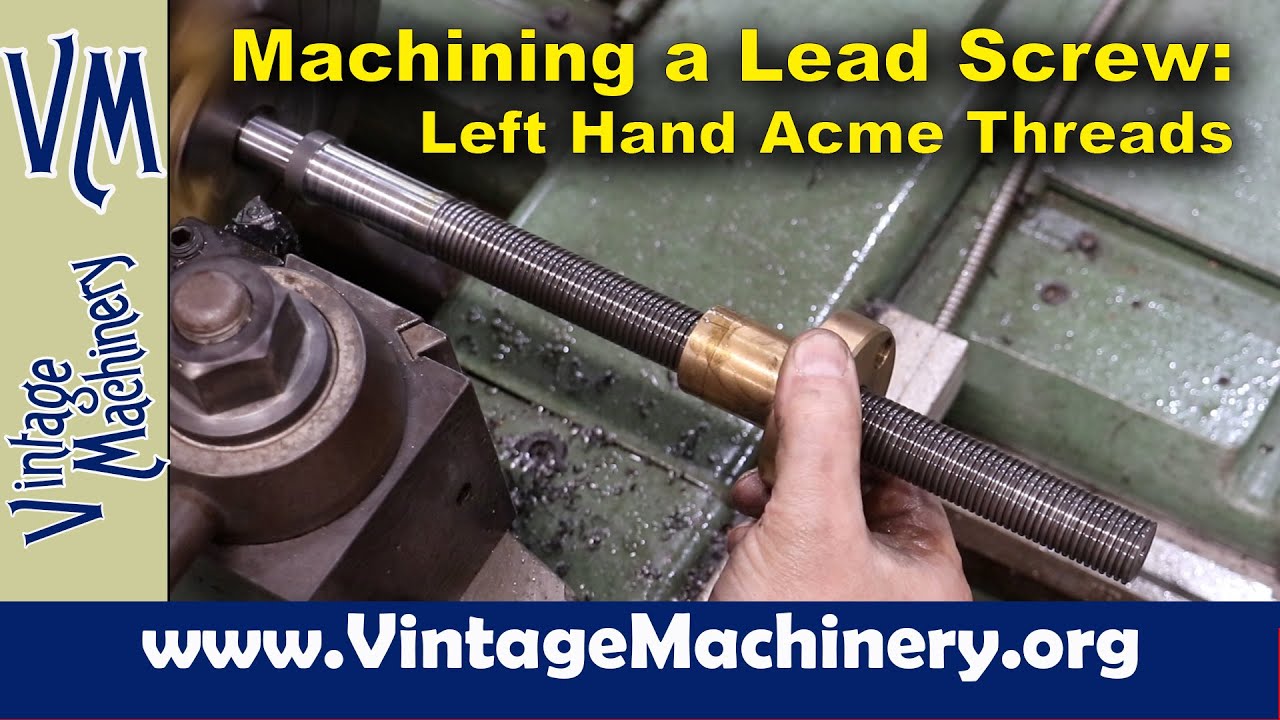The image is a detailed tutorial guide for machining a lead screw with left-hand Acme threads, featured on VintageMachinery.org. The center of the photograph prominently showcases a close-up of a man's right hand, visibly dirty and greasy, holding a silver lead screw with blackened threads. He appears to be threading a brass or gold-colored nut onto the screw, set against a backdrop of a grimy, metallic workshop environment.

A beige vertical banner on the left side of the image bears the blue-lettered logo “VM” and the words “Vintage Machinery.” Across the top, in a bold yellow font, are the words "Machining a Lead Screw: Left-Hand Acme Threads." At the bottom, a blue banner with white text clearly displays the website address, www.vintagemachinery.org. This comprehensive and instructional poster provides visual and textual elements to assist users in understanding the specialized process described.